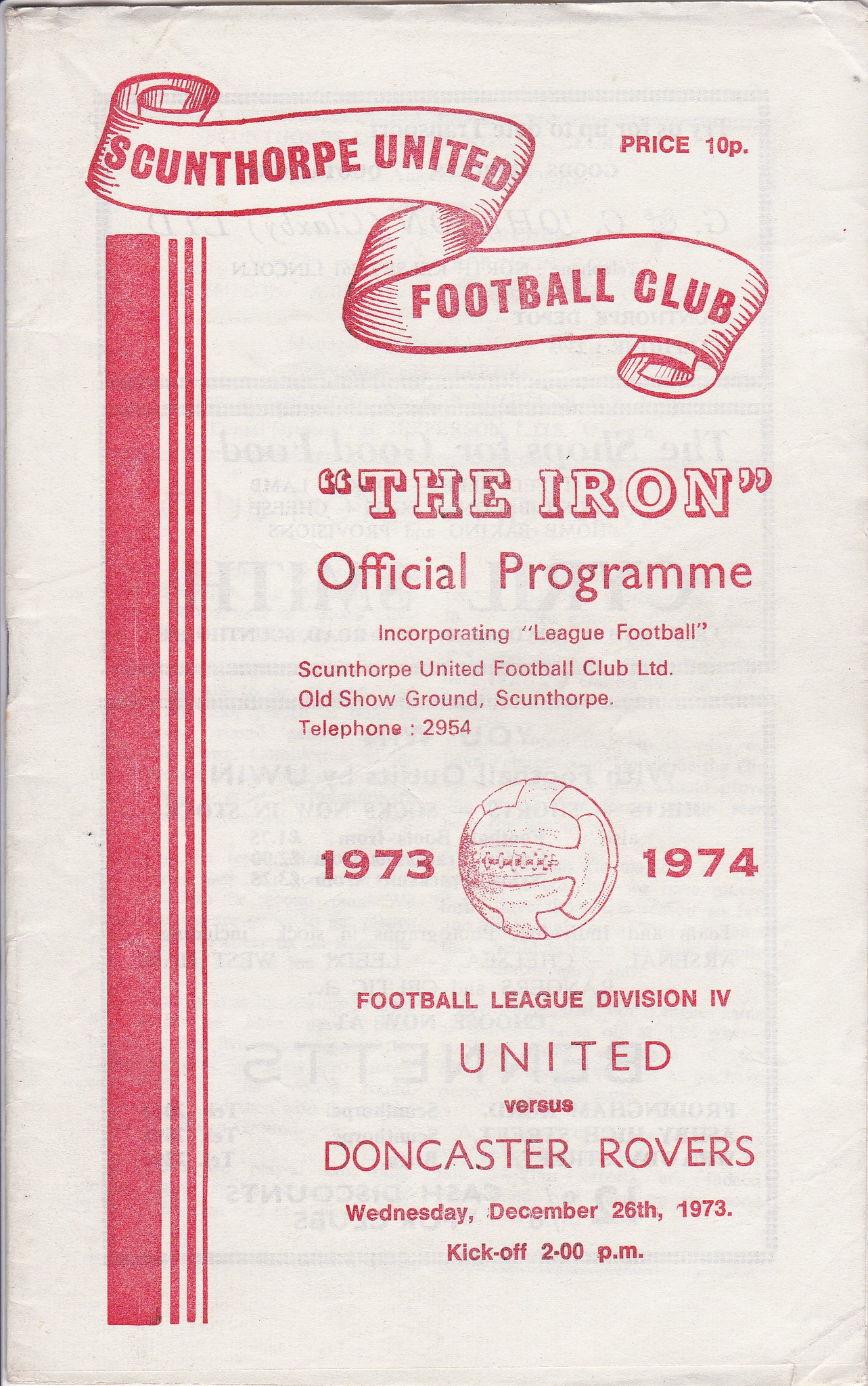The image features the front cover of an official soccer program for Scunthorpe United Football Club, dated December 26, 1973. The program has a white background with prominent red lettering. At the top, there is a banner displaying "Scunthorpe United Football Club." Just below, it reads "The Iron Official Program Incorporating League Football," followed by the details of the club: "Scunthorpe United Football Club Ltd, Old Show Ground, Skunthorpe, Telephone 2954." The cover lists the date range "1973-1974," and between these dates lies an illustrated red soccer ball. Additional text indicates that this is for the Football League Division Four match, featuring United vs. Doncaster Rovers, with the kickoff scheduled for Wednesday, December 26, 1973, at 2 p.m. The price of the program is marked as 10 pence.